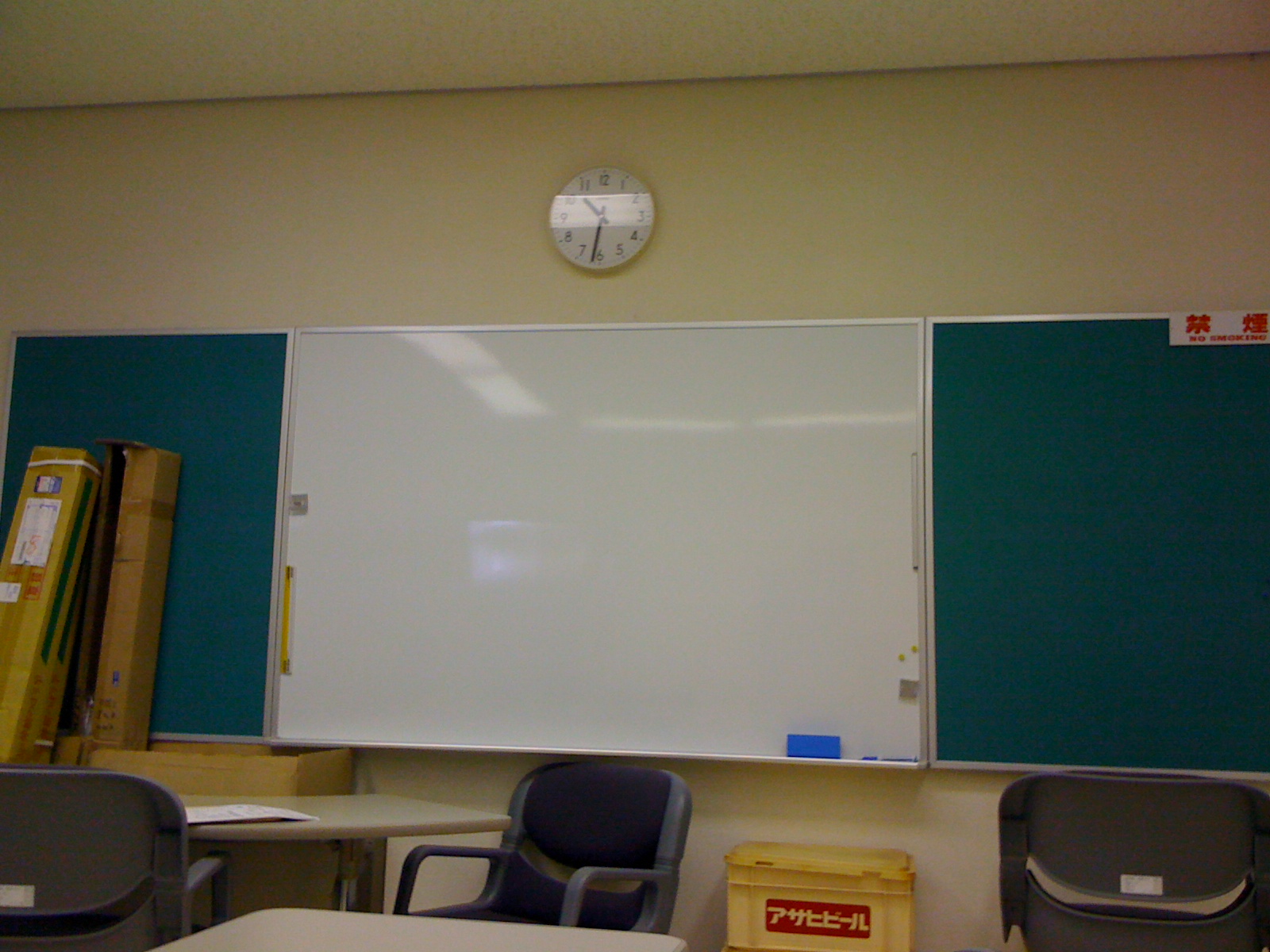The image depicts a classroom with a tan, off-white wall. The focal point is the teacher's area, highlighted by a whiteboard flanked by two green bulletin boards. Above the whiteboard, there's a clock showing the time as slightly past 10:30, although it is partially obscured by glare. A "No Smoking" sign with foreign characters is faintly visible on the right bulletin board. The floor is arranged with tables and chairs, including a beige table and seating positioned towards the whiteboard. On the left side, several tall boxes, possibly containing furniture, rest against the board, while a slightly open package and a yellow crate with foreign writing sit on the floor towards the right. A blue eraser is also noticeable on the bottom-right edge of the whiteboard.